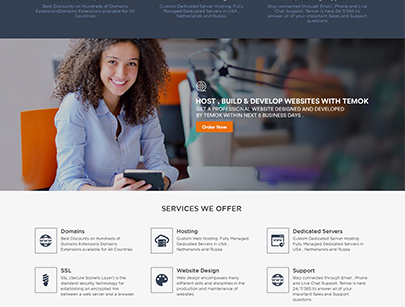This image is a detailed screenshot from the TMock website, a platform dedicated to hosting, building, and developing websites. 

At the top of the image, there's a blue banner with very small, unreadable text. Directly below this banner, a background image features a woman with curly hair, wearing a blue long-sleeve shirt. She is sitting comfortably in an orange chair at a desk, holding a notebook and sporting a large smile. 

To the right of this image, the scene becomes darker and blurrier, revealing a lamp and a person in the distant background. Overlaid on the image in white font are the words, "Host, build, and develop websites with TMock. Get a professional website designed and developed by TMock within the next five business days." 

Beneath this text, an orange button stands out with the call-to-action, "Order Now."

Further down, the image transitions to a white background featuring the heading, "Services We Offer." Listed under this heading are service categories such as Domains, SSL, Hosting, Website Design, Dedicated Servers, and Support, each accompanied by a small text description and a corresponding icon.